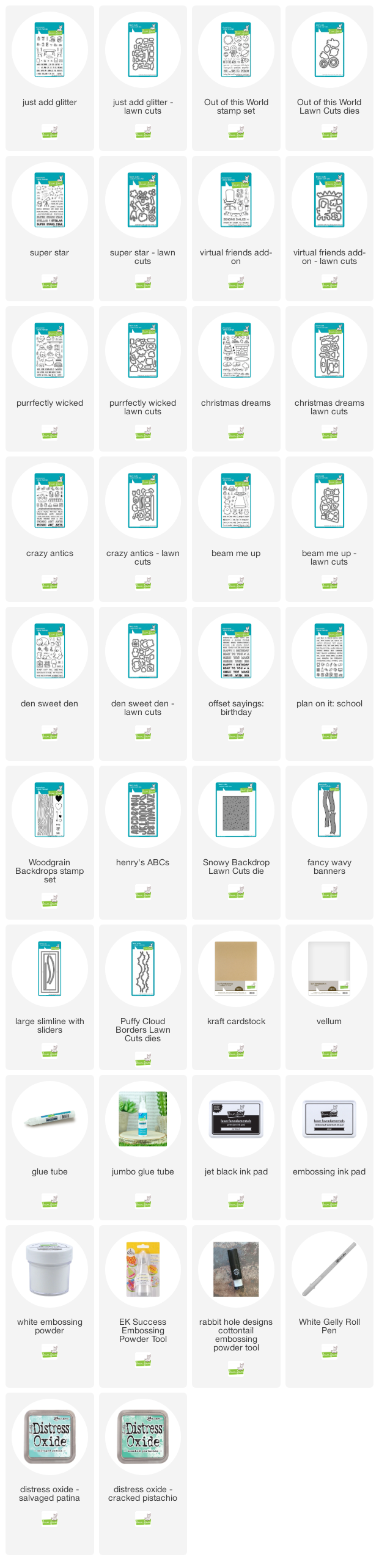The screenshot showcases a neatly organized grid with light gray squares, separated by thin white lines, arranged in a 4 by 10 formation. Each square contains product names, running horizontally and vertically. 

In the first row from left to right, the labels read: "Just Add Glitter," "Just Add Glitter Lawn Cuts," "Out of This World Stamp Set," and "Out of This World Lawn Cuts Dies."

The second row includes: "Super Star," "Super Star Lawn Cuts," "Virtual Friends Add-on," and "Virtual Friends Add-on Lawn Cuts."

The third row lists: "Perfectly Wicked," "Perfectly Wicked Lawn Cuts," "Christmas Dreams," and "Christmas Dreams Lawn Cuts."

The fourth row shows: "Crazy Antics," "Crazy Antics Lawn Cuts," "Beam Me Up," and "Beam Me Up Lawn Cuts."

The fifth row contains only one label: "Den Suite Den."

This detailed screenshot likely represents a catalog or inventory of crafting supplies, particularly involving stamps and die cuts.